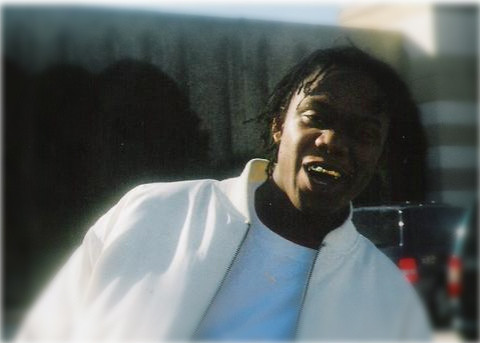This full-color outdoor photograph captures a young African-American man with short braided hair, sporting a big, open-mouthed grin that reveals a gold grill covering his teeth. He is dressed in a white jacket with a zipper, left open to reveal a plain white T-shirt underneath. His head is slightly tilted to the left, and he is illuminated by sunlight, which accentuates one eye while casting the other in shadow. In the background, one can discern blurred imagery of very tall buildings, some trees, and possibly traffic signs. The sky above is a clear blue. On the lower right corner of the image, two SUVs are vaguely visible. Adjacent to him, the backdrop features a metal wall with vertical lines, and to the left of his head, there’s a structure adorned with horizontal white stripes against a light green background.